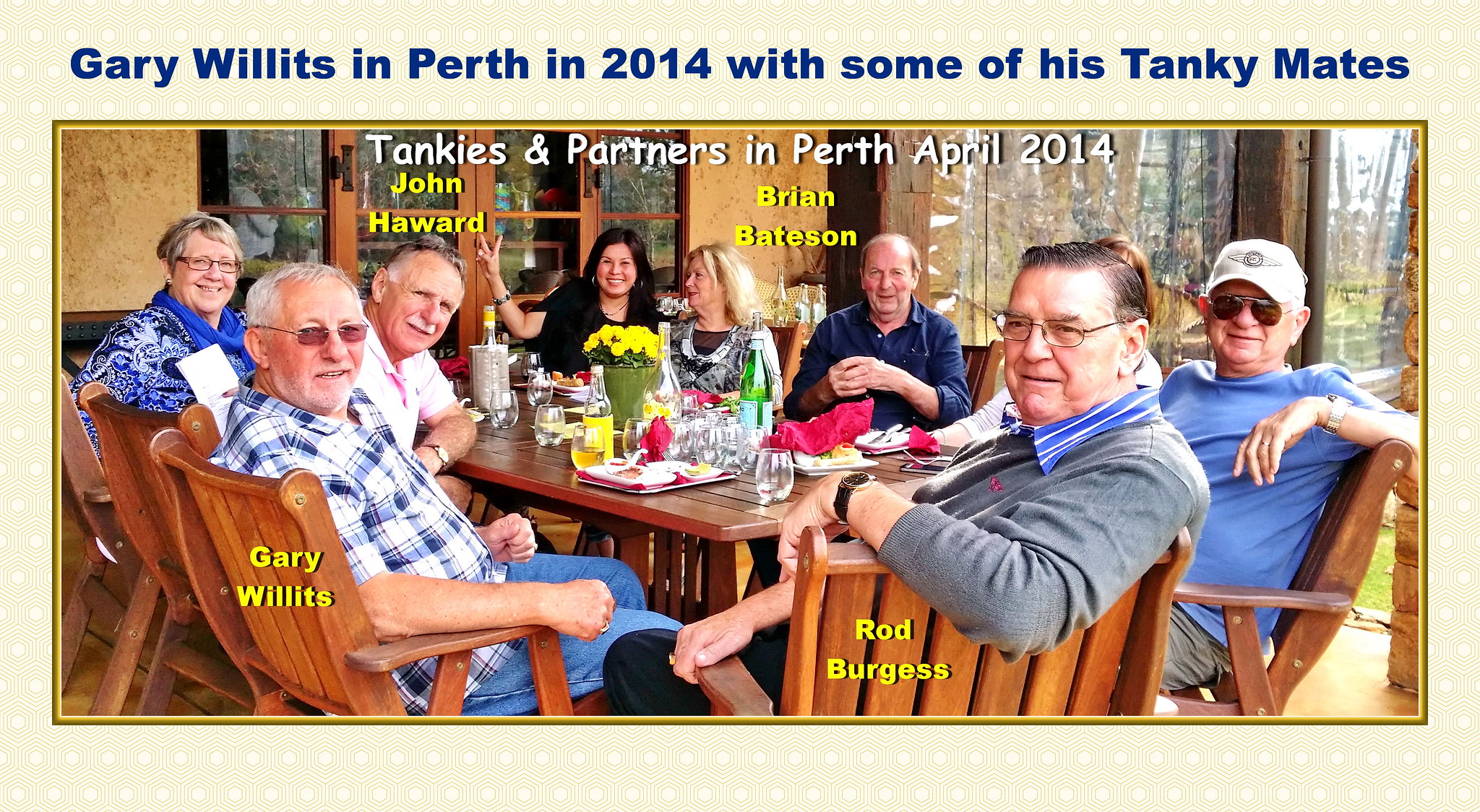The image captures a vibrant outdoor gathering of people seated around a wooden table adorned with food, drinks, and a bouquet of yellow flowers. The setting is bright and naturally lit, featuring a backdrop of trees, grass, and doors. At the top of the image, yellow and blue text reads, "Gary Willits in Perth, 2014 with some of his Tankie mates" and "Tankies and Partners in Perth, April 2014". 

From left to right, the attendees are identified with names in yellow text: a man in a blue and white plaid shirt, glasses, and sunglasses labeled as Gary Willits; a man in a white shirt with gray hair and a mustache leaning forward; a woman with short gray hair wearing glasses and a blue scarf; a woman with dark black hair in a black shirt holding a peace sign; next to her, a woman with blonde hair facing left; a man in a dark blue shirt with his hands in front of him; partially blocked, a man with glasses in a gray shirt, possibly wearing a gold watch; and another man in a blue t-shirt, cap, and sunglasses identified as Rod Burgess, with his arm over the back of the chair. Towards the back, another man, John Howard, leans in towards the table on the left, and Brian Bateson, with his hands together, is positioned at the back right. The entire image is framed by an intricate yellow border.